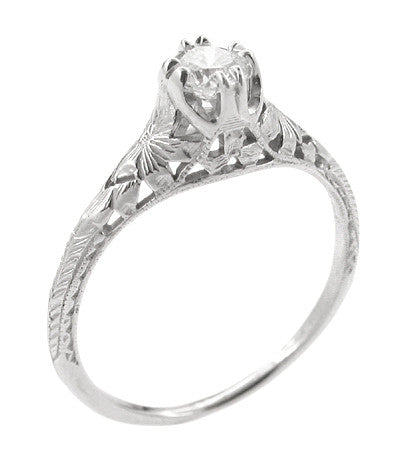This photograph captures a close-up image of a silver engagement ring against a pure white background, highlighting its intricate design elements. The ring, made of a silvery-looking metal that suggests but might not be actual silver, features a simple band that becomes highly detailed as it approaches the top. The lower part of the band is plain and thin, while the upper part showcases elaborate etchings, swirling patterns, and cutouts that resemble floral themes or starbursts. These cutouts add height and complexity to the design, culminating in an ornate, trident-like setting that holds a faceted diamond. The diamond is secured by eight prongs, and the overall craftsmanship includes delicate texturing and semi-intricate cutouts that give the ring a sophisticated and elegant appearance.